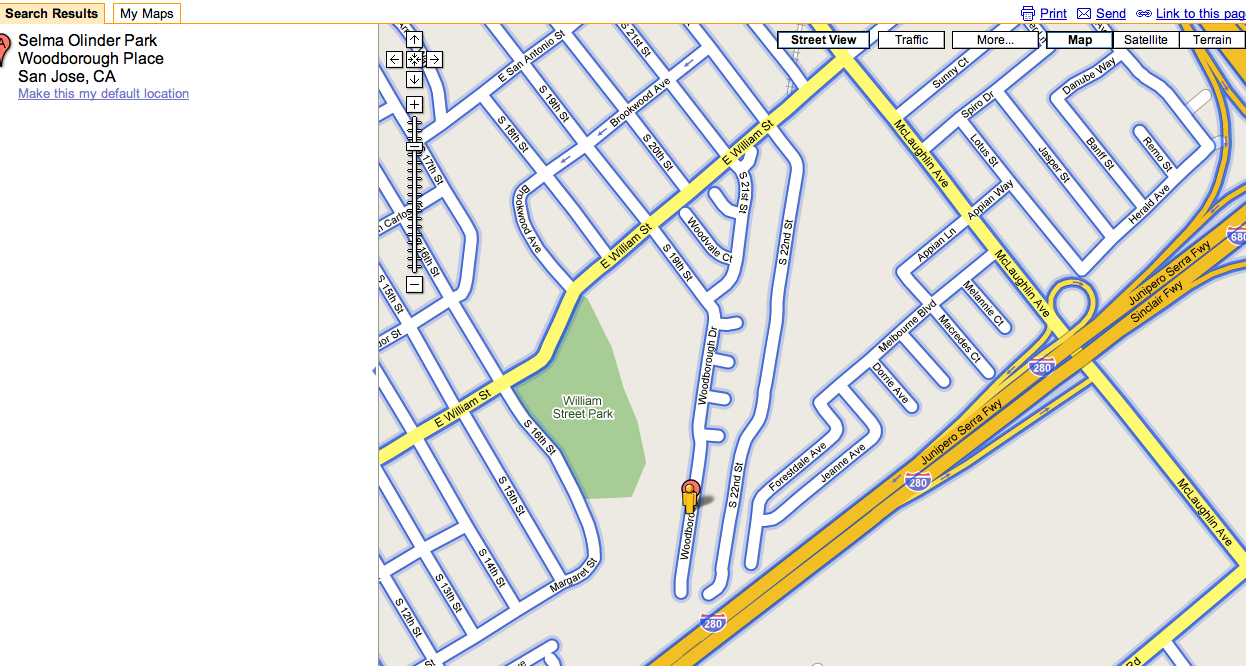**Caption:**

A map interface displayed on a tablet or laptop screen, showcasing detailed driving directions. The interface is in landscape orientation. On the left, a tab labeled "Search Results" is highlighted in red, indicating its active status, while an adjacent tab "My Maps" remains unselected in white. Below the highlighted tab, blue underlined text reads "Selma, Olinder, Park, Woodborough Place, San Jose, California," with a hyperlink offering the option to make this the default location.

In the upper right section of the interface, several icons are present: a printer icon for printing, an envelope icon likely for sending, and a mail icon which might link to the map or page, possibly in PDF format. 

The right half of the interface is dominated by a road map. A major road is marked in yellow or orange, indicating the specific route, while smaller roads are colored white. A green area represents a park. Street names are printed in black, and every visible street is labeled. An additional street features directional arrows, possibly denoting a one-way street. The map's background is light gray.

Control arrows for navigating the map (up, down, left, right) are located in the top left, accompanied by a zoom slider. The top right of the map hosts six selectable boxes: Street View (currently selected), Traffic, More..., Map, Satellite, and Terrain, allowing users to switch between different views.